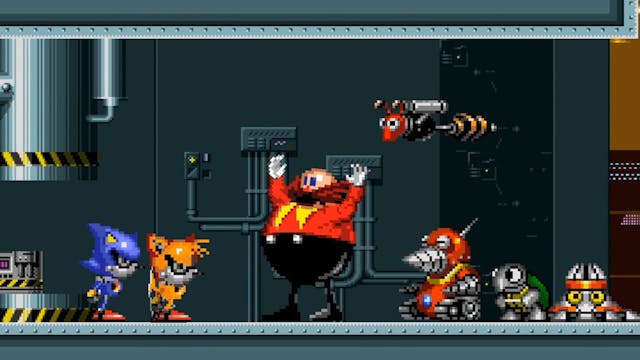The detailed caption for the image is:

This is a screenshot from the classic Sega Genesis video game, Sonic the Hedgehog. The 16-bit graphic showcase features several iconic characters lined up on a metallic surface that resembles a conveyor belt, indicative of a factory setting. In the center of the image stands Dr. Robotnik, a bald, rotund man with a large, bushy red mustache that extends beyond his head. He is wearing a red shirt with yellow details, black pants, yellow suspenders, and white gloves, with both of his arms raised above his head. To his left side, we see Sonic the Hedgehog, a small blue anthropomorphic hedgehog known for his distinctive orange shoes, and Tails the Fox, an orange anthropomorphic fox with similar footwear. Next to Robotnik stands a robot on gray tracks featuring a red body, a round red head, a gray antenna, and a drill on its face. Additional robotic enemies are visible as well, including a robotic bee, a turtle, and various other menacing metallic creatures, all of which are characters from the Final Egg Zone level in the game. The background presents a gray, industrial theme with machinery on the left side, enhancing the factory-like atmosphere of the scene.